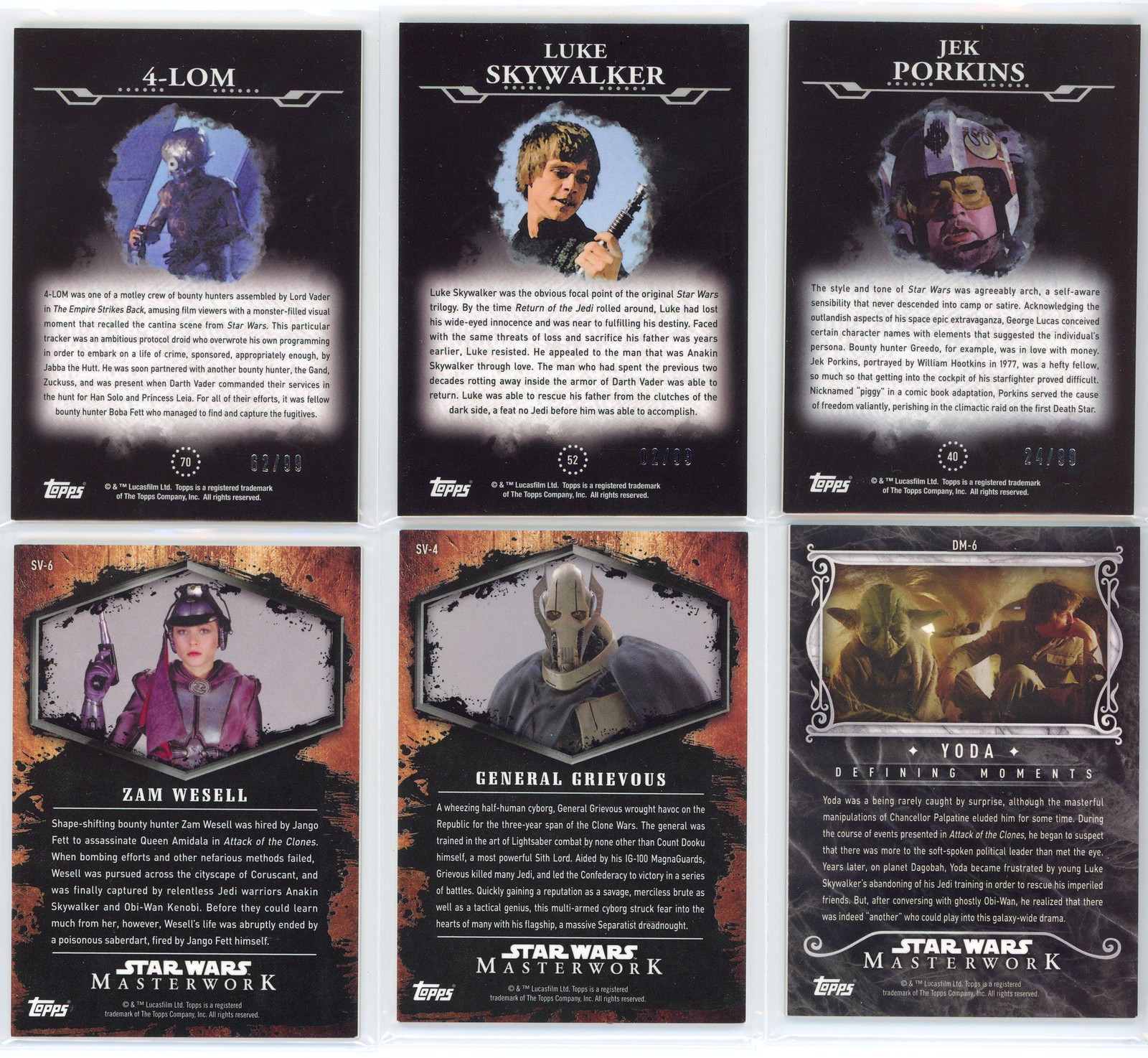The image is a detailed showcase of six Star Wars trading cards, arranged in a 3x2 grid. The top row features cards of Forlorn, Luke Skywalker, and Jack Porkins. Each of these cards presents the character's name at the top, followed by their picture, with general details about the character listed underneath. The backgrounds of these top row cards are predominantly plain black.

The bottom row includes cards of Zam Wessel, General Grievous, and Yoda. In contrast to the top row, these cards start with the character's image at the top, followed by their name, and details below. These bottom row cards are from the Star Wars Masterwork set, distinguished by their more intricate and colorful backgrounds, including bronze accents for Zam Wessel and General Grievous, and additional vibrant coloring for Yoda. Overall, the arrangement and design emphasize the detailed and collectible nature of these character cards, highlighting their importance in the Star Wars universe with a diverse palette of colors ranging from earthy hues to bright highlights.